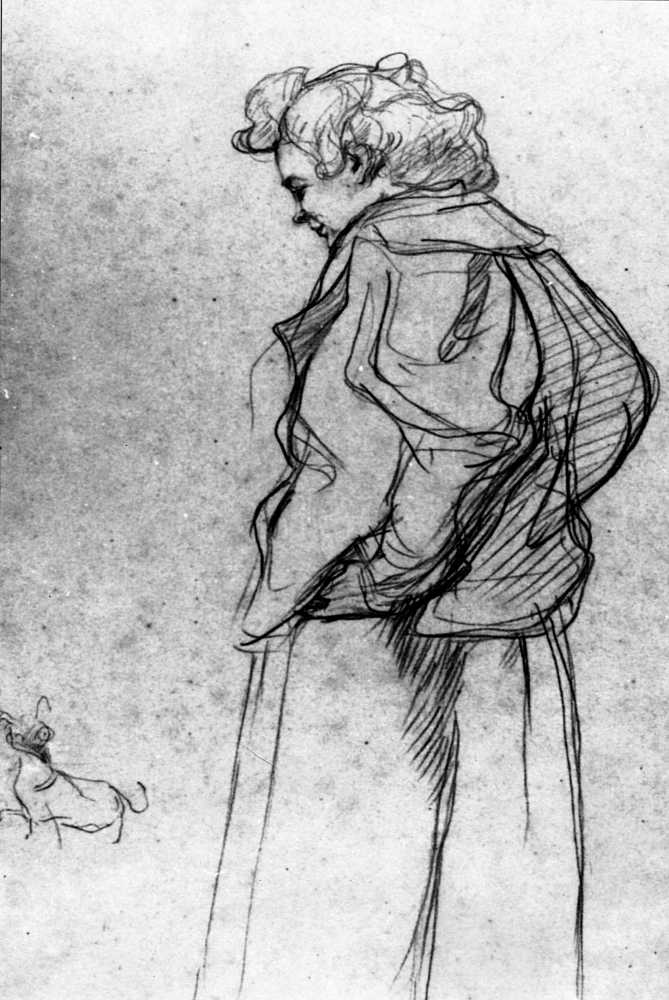This detailed black and white sketch titled "Madame Palmieri with her Dog" by Toulouse-Lautrec, created in 1897 in post-impressionism style, depicts a woman in her mid-70s standing and looking down to her left at a small dog with an elongated body and small head. The woman, viewed from behind in a side profile, has a poofy section of hair at the top which does not extend far down her neck. Dressed in a bulky blouse or jacket and a long skirt that reaches her feet, she is somewhat heavyset and has her hands on her hips, though the exact positioning suggests they might be in her pockets or in front of her. She has a stern expression on her face. The sketch is in black against a grayish white background, with the woman occupying most of the vertical space. The small dog is placed at the bottom left, indicated with minimal, simplistic black strokes.